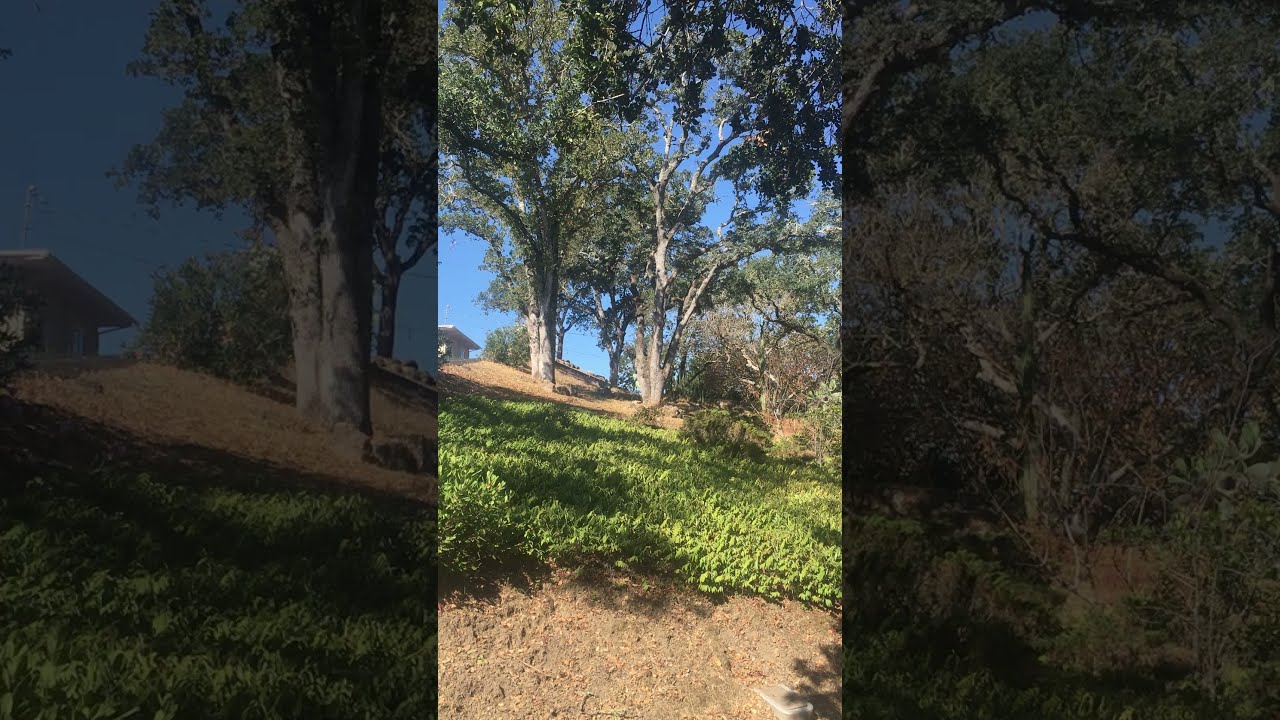The image is divided into three equal vertical sections, with the left and right sections appearing grayed out, contrasting the vivid central section. The central section displays a sunny, dry woodland scene leading up a hill. At the bottom, patches of dry soil and leaves transition into green grass and vegetation, which are dotted with sunlight and shadows. Tall trees with white, gray, and silver bark rise with branches of green leaves. In the background, a blue, cloudless sky peeks through the foliage. A white house with an angled roof is situated at the top of the hill on the left, partly obscured by bushes and hedges. The landscape suggests a residential neighborhood.